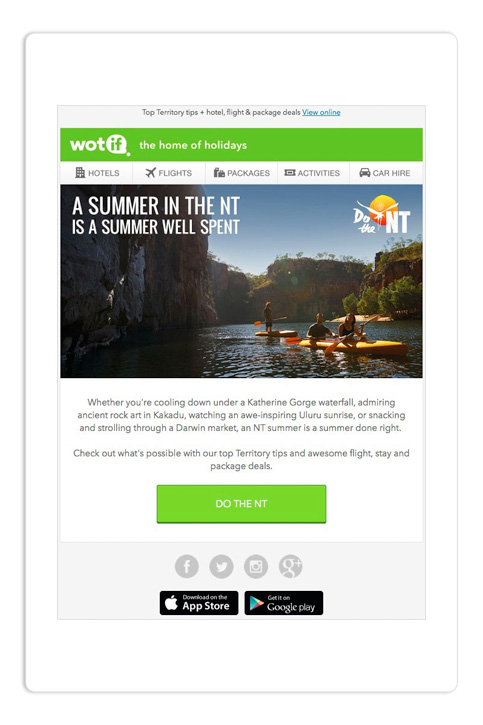### Descriptive Caption for the Image

The image appears to be a screenshot of a promotional website. The entire image is vertically rectangular and framed by a thin light gray border. The background is predominantly white. 

Near the center, but slightly lower from the top, is a section also outlined with a thin gray border. This section is topped by a narrow gray horizontal strip containing the text "Top Territory Tips plus Hotel Flight and Package Deals View Online."

Beneath this strip, a green section features prominently. On the left of this green section, the words "What If" are displayed in white, followed by the words "WOT" written in green letters within a white bubble, and then the phrase "The Home of Holidays" in white.

Directly below this, a white horizontal area contains clickable buttons labeled: Hotels, Flights, Packages, Activities, and Car Hire.

Further down, there is a striking image of what appears to be a canyon. The canyon features rock cliffs and what looks like a river flowing through it. The river has several people engaging in water activities: a couple paddling in a kayak, and a man standing on a paddleboard with a paddle. Surrounding the cliffs, both at the top and bottom, are scattered trees.

Below the image, text reads: "Whether you're cooling down under a Katherine Gorge waterfall, admiring ancient rock art in Kakadu, watching an awe-inspiring sunrise, or snacking and strolling through a Darwin market, an NT summer is a summer done right. Check out what's possible with our top territory tips and awesome flight, stay, and package deals."

A large rectangular lime green button labeled "Do the NT" in white letters is prominently displayed below this text.

At the bottom, a light gray area features symbols for various social media platforms, including Facebook, X (formerly Twitter), Instagram, and Google Plus. Below these icons are two additional buttons for accessing the website via the Apple Store and Google Play.